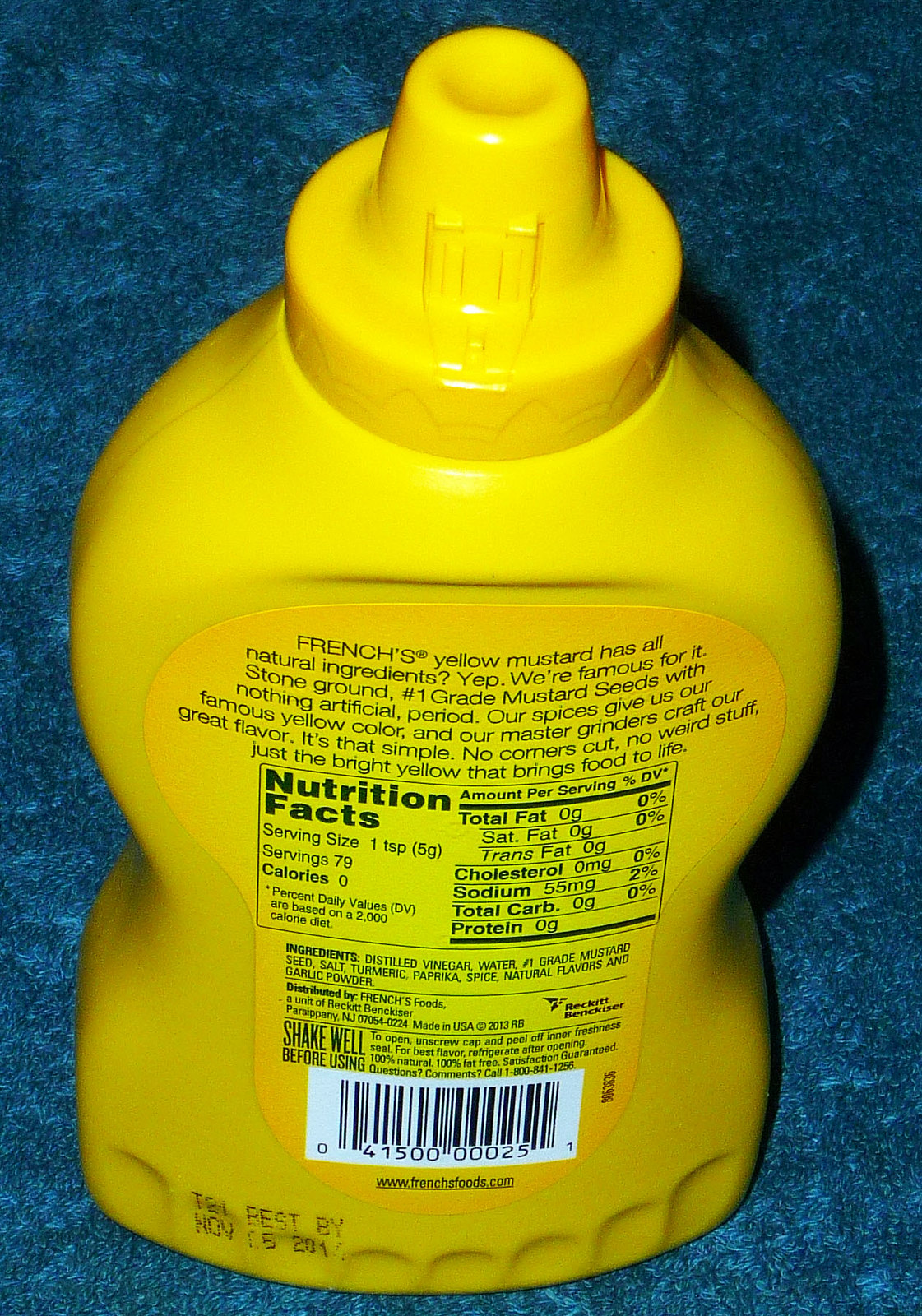The image depicts the back of a French's Yellow Mustard container, prominently showcasing some of the text on its label. The text reads: "French's Yellow Mustard has all natural ingredients. Yep, we're famous for it. Stone ground, number one grade mustard seeds, with nothing artificial, period. Our spices give us our famous yellow color, and our master grinders craft our great flavor." Positioned at the bottom of the bottle, the bar tag is visible. The container rests on a blue carpet or rug. The "Best if used by" date is marked as November 15th.